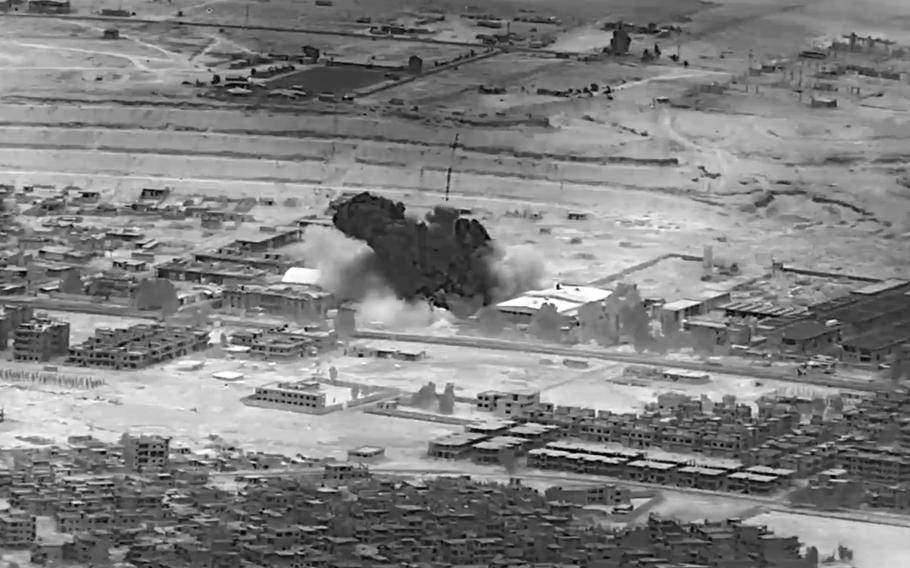The black-and-white photograph, potentially a wartime image, provides a distant, aerial view of an industrialized area densely packed with what appear to be hundreds of buildings. In the center of the frame, there's a clear point of impact, likely from a drone strike, marked by a large black blob of smoke and dust, with lighter smoke surrounding it. This explosion has hit one of the buildings, and the aftermath is evident amidst the closely packed structures. The image, although a bit blurry, captures the stark contrast between the impacted area and the rest of the untouched buildings. The background showcases what seems to be roadways and a small community or village, adding to the sense of scale and devastation within the industrial area.